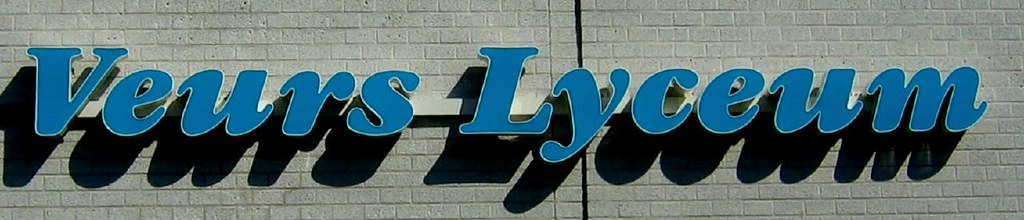This photograph captures a store sign prominently displayed on the exterior of a light gray brick building. Bathed in bright sunlight, the sign features individual 3D letters in a striking medium blue color, mounted on a sleek silver horizontal bar. The sign reads "VEURS LYCEUM" in italicized print, with the sun casting distinct shadows of the letters onto the building facade below, adding a dynamic and engaging visual element.